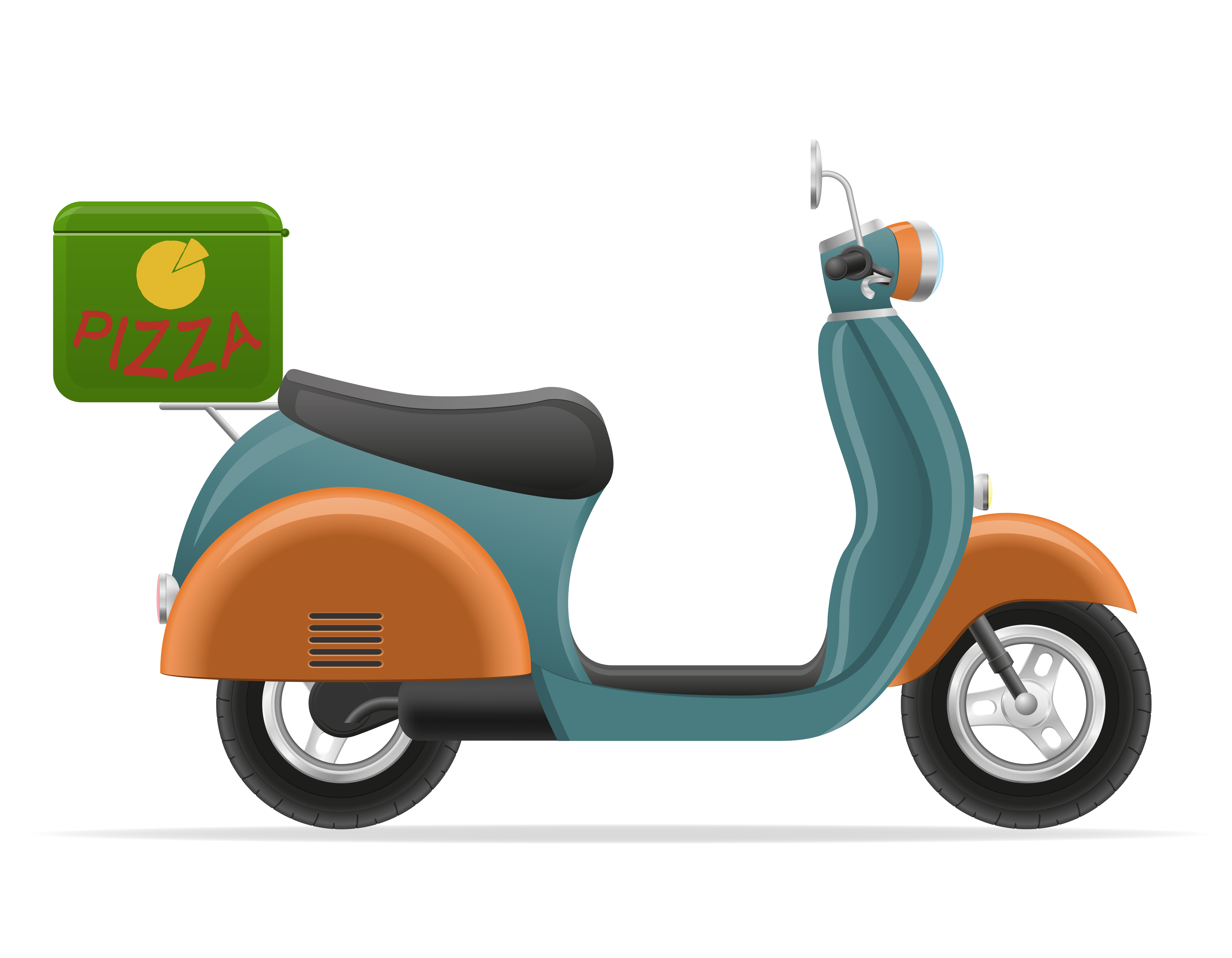The image depicts a vector graphic clipart of a side-view scooter with a predominantly teal color. The scooter, facing right, features black and gray wheels with silver hubcaps, a black seat, and a black handlebar accompanied by a gray mirror. A green box specifically designed for pizza delivery is mounted on a gray stand behind the seat. This green box has a prominent yellow circle with a yellow pizza slice illustration and the word "pizza" written in bold red letters beneath it. Additionally, there is a gray shadow under the scooter, emphasizing its form.